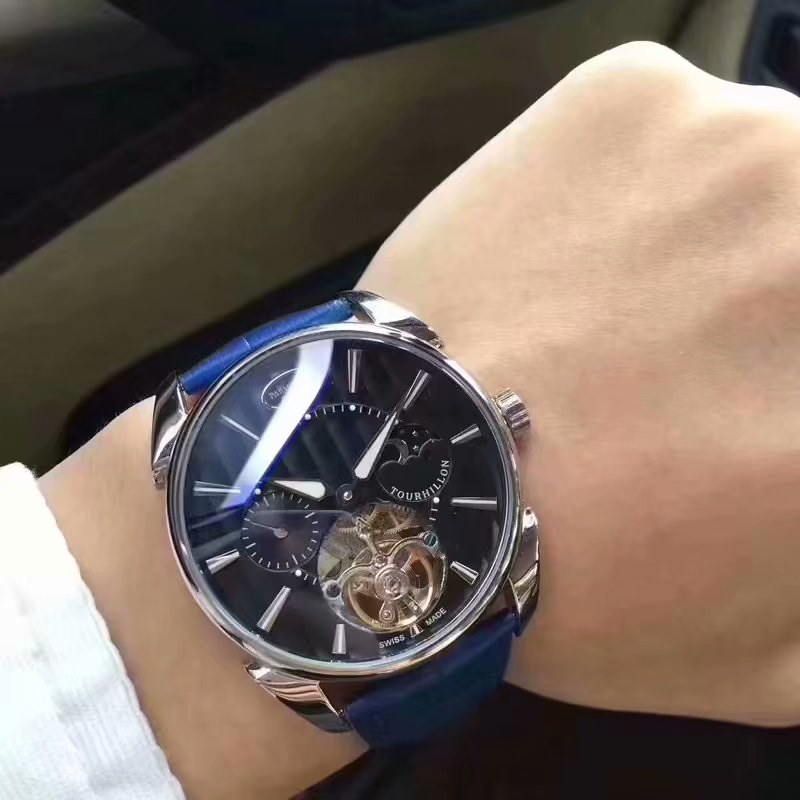This real-life photograph showcases a person's wrist adorned with a striking wristwatch. The individual, who has light skin, holds their hand in a partially clenched fist, slightly extending beyond the image's border. The wristwatch features an elegant blue silky strap that contrasts beautifully against the skin tone. 

The watch face is large and circular, encased in a chrome frame with a reflective cover that catches the light. Within the watch face, an intricate clock mechanism devoid of traditional numbers is visible, with delicate metal bars marking the hours. The watch hands are slender and white, positioned at 10:10. Additional smaller dials and mechanical elements are situated at the bottom, revealing the watch's inner workings.

At the top center of the watch face, a logo is present but partially obscured by glare. The wrist extends from a sleeve that has a unique wavy cuff, distinguishing it from a typical design. The background beneath the hand is somewhat ambiguous, featuring a khaki fabric with dark brown edges surrounded by mostly black areas, adding a subtle touch of mystery to the scene.